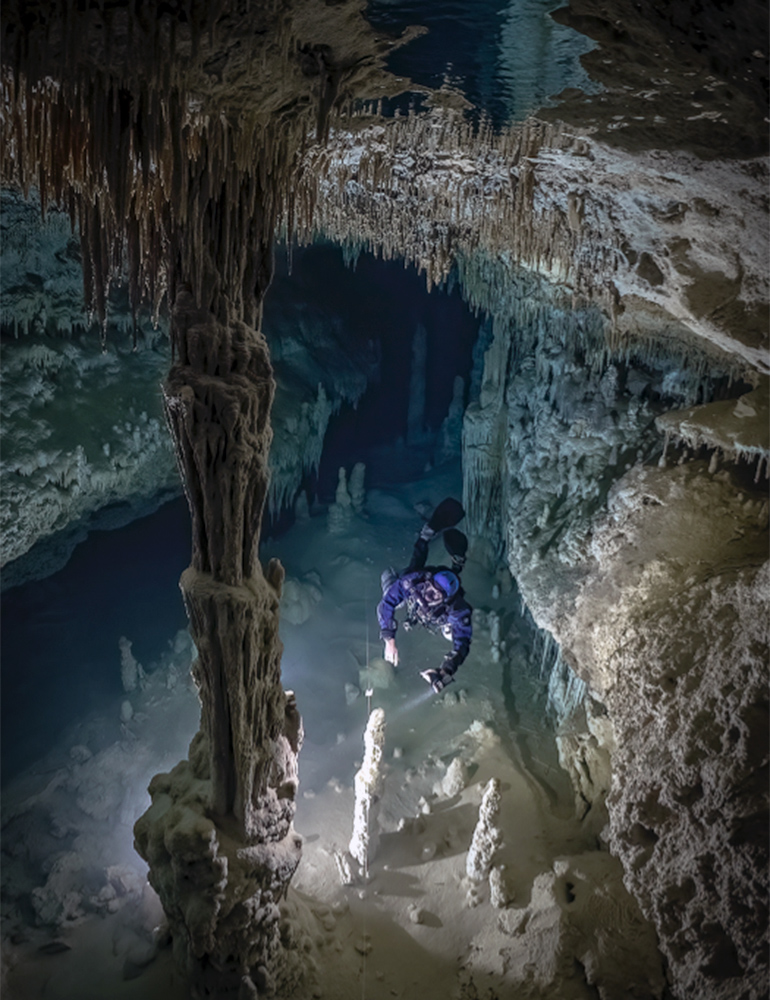The photograph captures an underwater diver exploring a unique and exotic underwater cave. The diver, dressed in a blue scuba suit with black fins, navigates the clear waters while holding a flashlight in their left hand, illuminating the cavern around them. Reflective surfaces create an almost mirror-like image where the ceiling and floor seem to blend together, confusing the perspective. The cave's walls and floor showcase a range of colors including gray, brown, and white, adorned with stalactites and stalagmites, as well as coral reef-like structures. The diver appears to be examining a large pillar within the cave, intent on their journey. The water's clarity makes it appear as if the diver is floating mid-air, adding to the surreal atmosphere of this captivating scene.